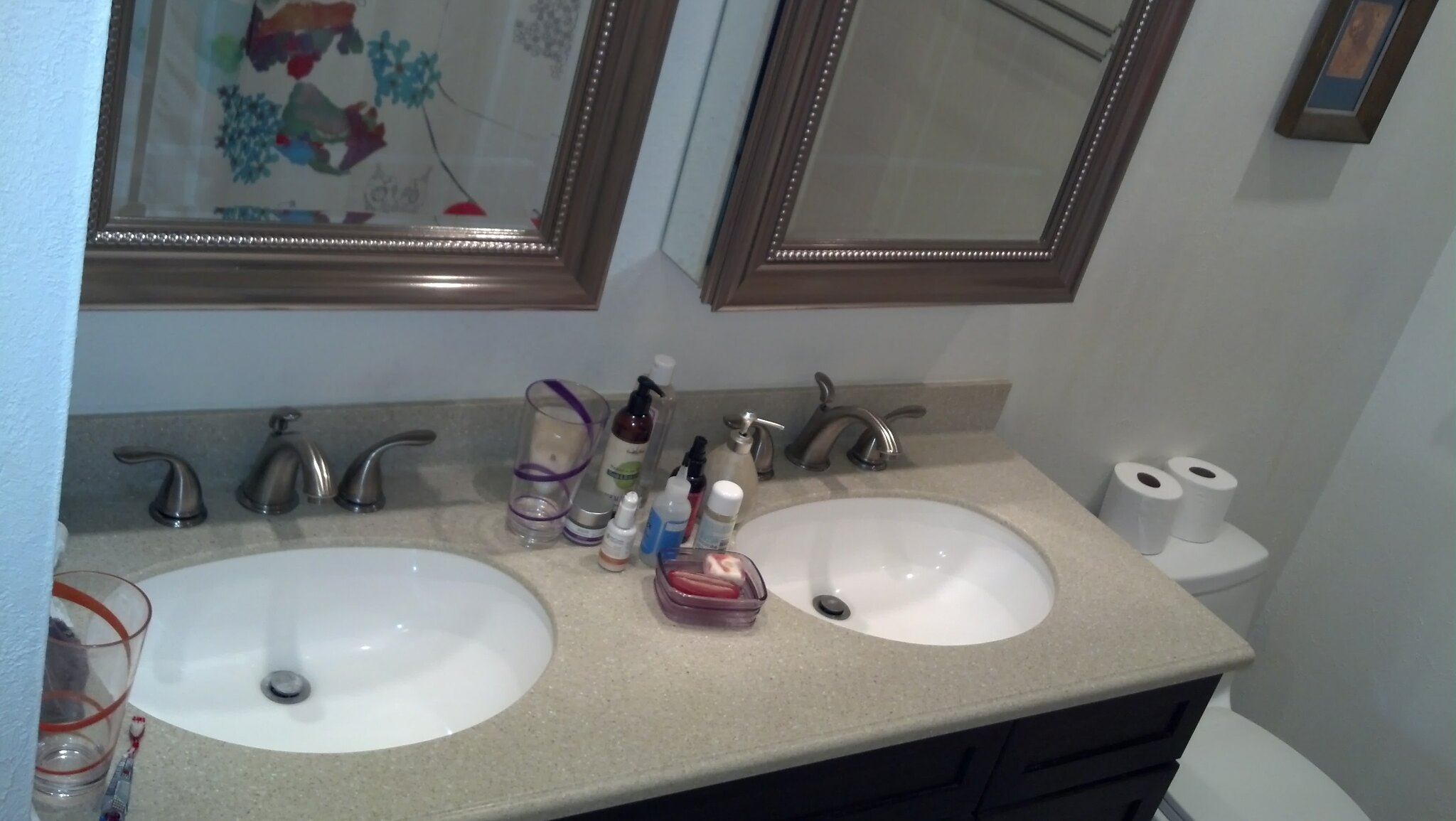This photograph showcases a master bathroom in a home, featuring a double sink setup indicative of a "his and hers" design. The left side of the image captures the edge of one of the sinks, extending approximately three-quarters of the way across the frame, where it meets a toilet adorned with two rolls of toilet paper. Above the toilet, a small piece of decorative art adds a touch of personalization to the space.

The vanity area boasts two mirrors positioned above the sinks, reflecting the shower curtain, which implies that the shower is situated opposite the sinks rather than next to the toilet. The countertop between the sinks is dotted with various toiletries, including soap pumps, contact lens solution, and other everyday essentials, providing a practical yet cluttered feel. In the bottom left-hand corner of the image, an organizer mounted on the wall appears to contain additional bathroom necessities, contributing to the room's overall functionality and convenience.